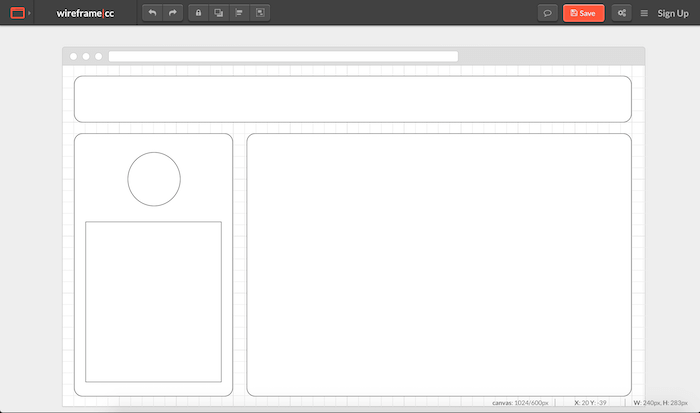The image depicts a computer screen displaying the interface of a web application titled "Wireframe CC," evident from the black header at the top of the screen. On the far left of the header, there is a prominent red rectangle which could presumably be a logo or a key indicator. 

On the upper right-hand corner of the header, a sequence of functional buttons is visible, listed as follows from left to right: a search bar button, a save button, a share button, a menu button, and a sign-up button. Adjacent to the title "Wireframe CC" within the header, there are additional buttons, including a back button, a forward button, a lock button, and a fullscreen button. The remaining buttons in that section are not clearly distinguishable.

The main content area of the screen is set against a gray background, with a graphical interface superimposed. A large, white, rounded rectangular strip spans across the top portion of this interface. Below this strip, there are two vertically-aligned, different-sized rectangles. The left rectangle is narrower and contains a small circle at its top, followed by a smaller rectangle directly beneath it. 

The right rectangle, significantly wider and about two to three times the size of the left rectangle, is conspicuously blank, filled solely with a plain white color absent of any additional elements or text.